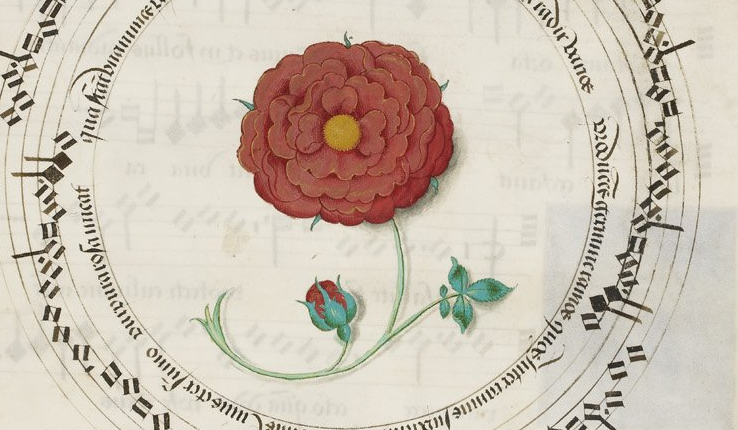This image is a detailed illustration on white paper, featuring a lush red flower with a yellow center prominently in the middle. The flower is intricately drawn with layered petals forming a lush bloom. Attached to the green stem, which curves elegantly, are several light green leaves and a smaller budding flower showing a hint of red. Encircling this flower is a large circle with words written in black, possibly in another language. Surrounding this central circle are four to five additional concentric lines. Along these lines are slightly rounded shapes resembling music notes, reminiscent of old shape-note music notation. The entire composition is detailed and complex, combining botanical illustration with elements of decorative and textual design.